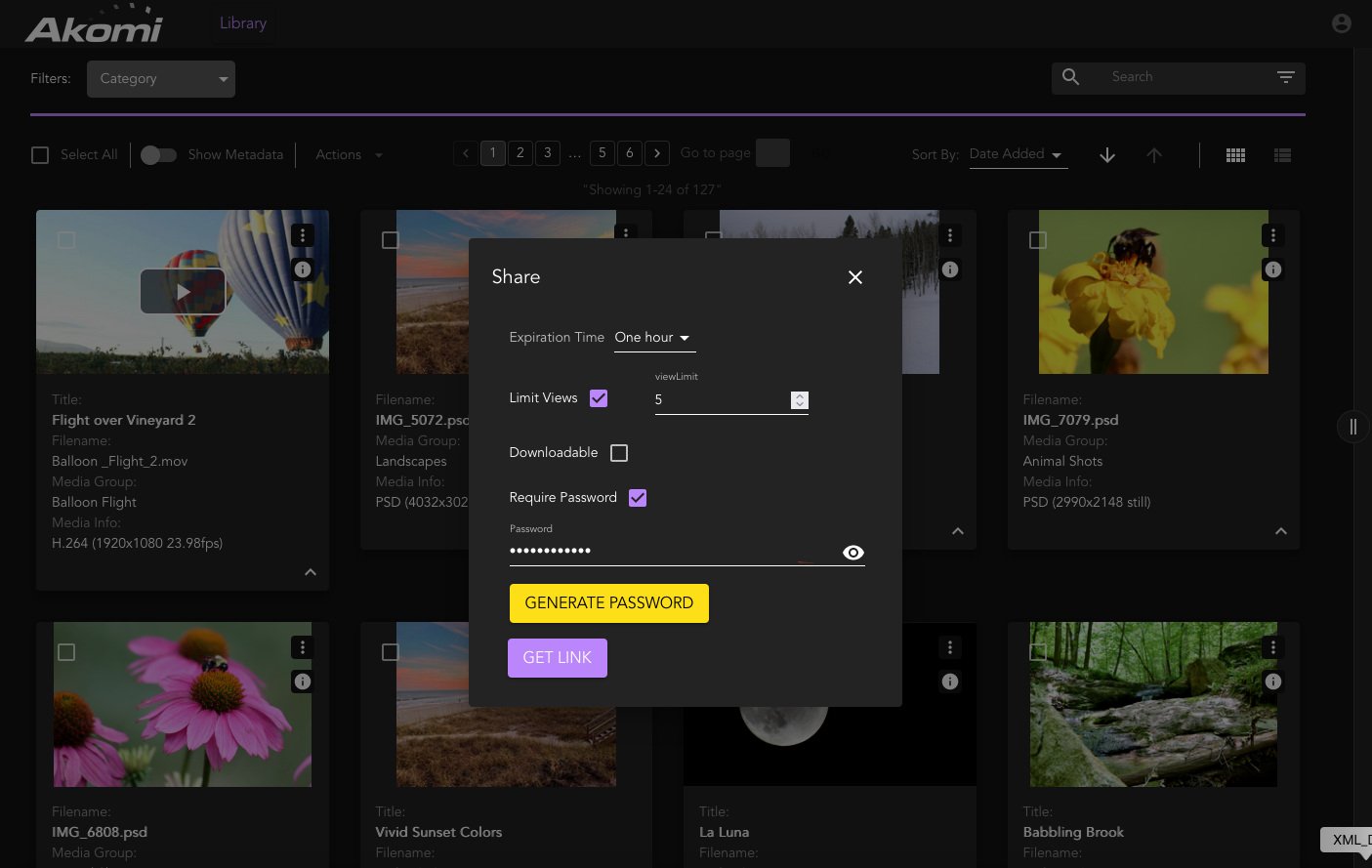The image depicts a digital interface with a primary focus on a rectangular pop-up window centered against a predominantly black background. This rectangular pop-up features white text and is bordered with soft edges. At the top of the pop-up, the word "Share" is prominently displayed in white font, flanked by two 'X' icons on the top-left and top-right corners, presumably to close the window.

Directly below, there are multiple options accompanied by checkboxes. Firstly, "Expiration Time: 1 hour" is listed. Then, there is the "Limit Views" option, which is checked with a black checkmark inside a purple box. The "Downloadable" option remains unchecked, while the "Require Password" option is checked, also in a purple box with a black mark. Beneath this, a password field displays an already entered password. An orange box labeled "Generate Password" sits below this section.

At the bottom of the pop-up window, a prominent purple box with white writing instructs users to "Get Link."

The background beneath the pop-up showcases a broader page featuring a grid layout of eight individual images. These images appear to be part of a gallery, with navigation options indicated by a scroll-through mechanism for viewing additional pages. In the top-left corner of the overarching page, "Okomi" is written in white text next to a "Category" label. On the top-right side, a search function is available for user convenience.

Specifically, in the bottom-left slot of the image grid, an image of purple daisies is noticeable. On the bottom-right, there is a serene scene capturing a river flowing through a rocky forested area. The entire composition suggests a sleek, modern design aimed at facilitating easy sharing and browsing of digital content.